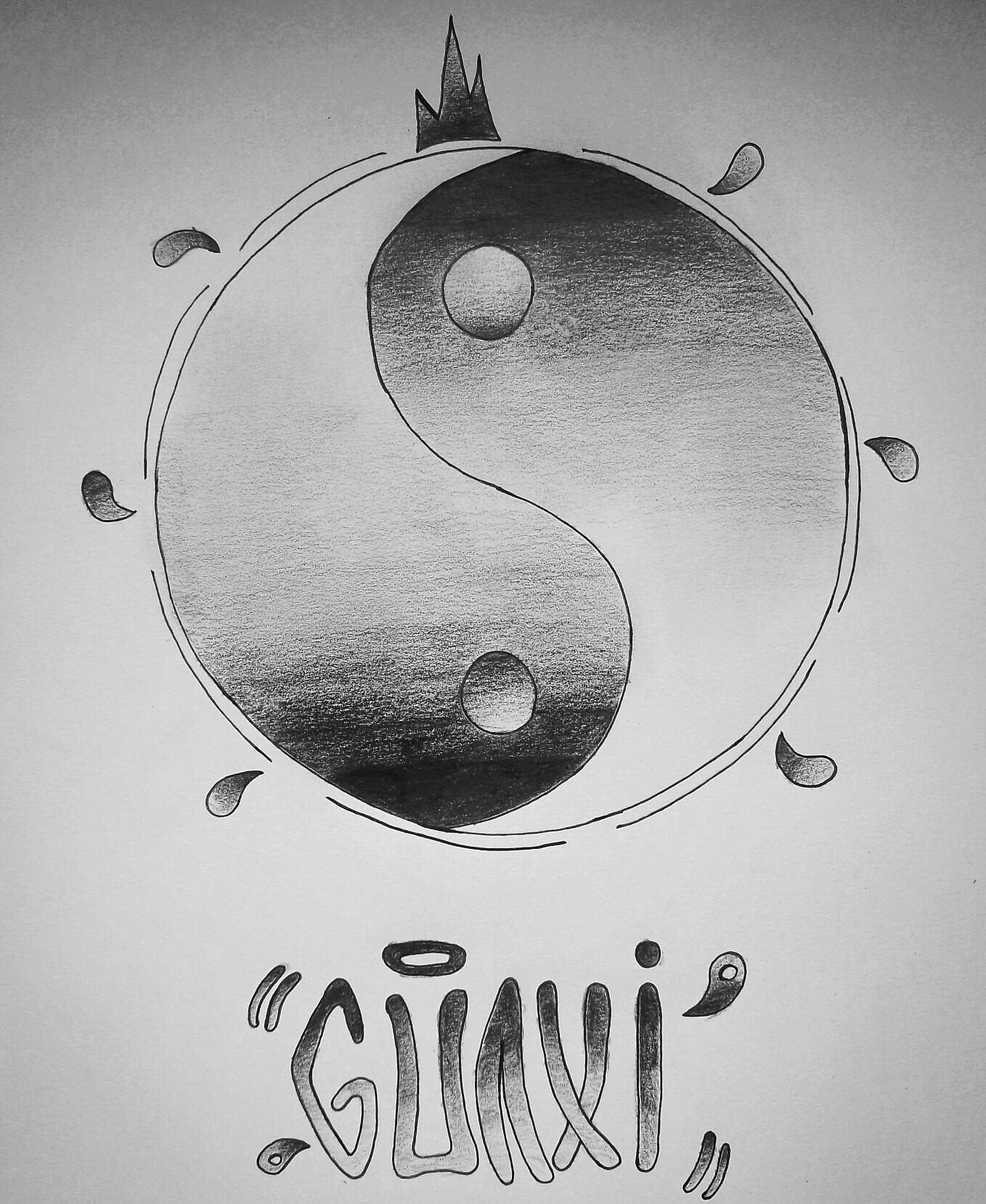The artwork features a vertical rectangular canvas with a predominantly black, white, and gray color scheme. At the center is an intricate rendition of a yin-yang symbol, but with a unique twist: both halves of the symbol transition from a slightly darker gray near the dots to a lighter gray as the curves extend. Notably, the dot on the right is marginally lighter than its counterpart.

Surrounding the yin-yang are six small, comma-like shapes dispersed evenly along the left and right sides, resembling sweat beads or water drops. Additionally, an outer circle encircles the yin-yang, drawn with a thin black line that is intermittently broken, from which more water drop shapes emerge.

Crowning the top of this composition is a trio of jagged, spike-like shapes that collectively resemble a mountain peak or shark fins. Just below the yin-yang symbol is the word "GUAXI," written in a dull black font. The 'A' in "GUAXI" is distinctively missing its middle horizontal line, and the 'X' appears to merge at the lower half rather than at the center. Above the letter 'U' is a small halo, further ornamented with additional brackets and commas.

Overall, the piece offers a detailed and meticulously designed take on traditional symbolism with modern and abstract elements integrated throughout.